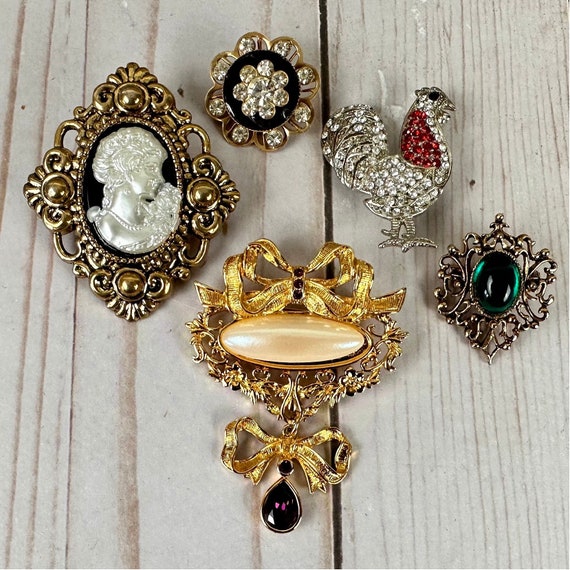This image depicts five intricately designed antique pins arranged in a diamond formation on a rough, unpainted wooden surface, reminiscent of a picnic table. From the left, the first pin features a pearl-like sculpted portrait of a woman against a black background, encased in a gold frame that resembles a locket. Next, a circular pin bursts with diamonds at its center and outer edges, echoing the look of a sunflower. The third pin showcases a dazzling rooster encrusted with white crystals and accented with red gems. Moving rightward, an elaborate floral brooch centers around a vibrant emerald, radiating gold branches set with white gems. Finally, the bottom piece is an opulent, golden pin adorned with two bow-like ornaments; the first is above a pearly beige stone, and the second, draping below, highlights a dark purple gem. The varied textures and rich details of these vintage pins contrast beautifully against the rugged wooden backdrop, giving a sense of timeless elegance and charm.